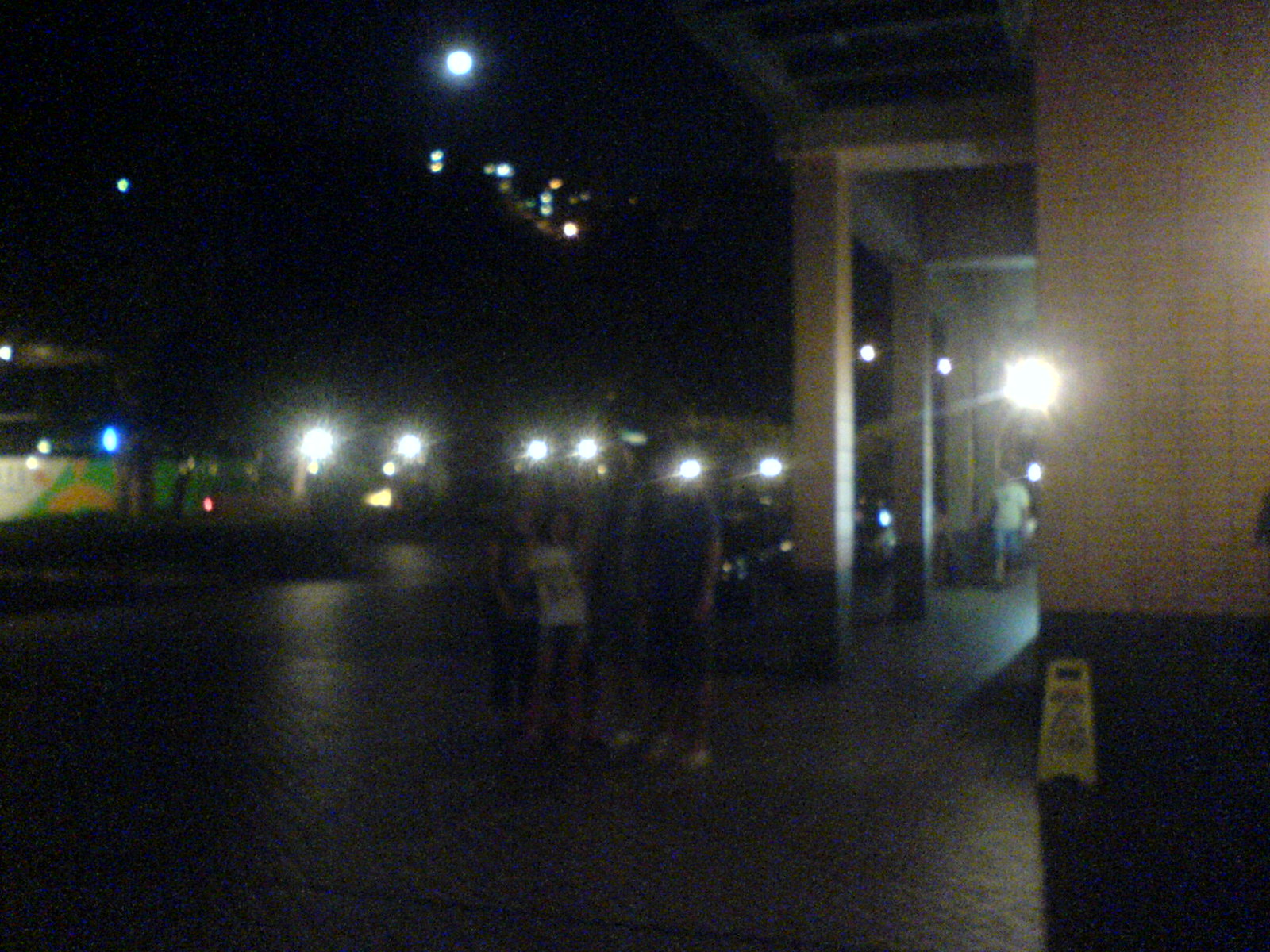This is a blurry nighttime photograph taken outside a white and black brick building, possibly a bank, club, or bar. The structure features tall columns that extend out into an awning and tiling along its sides. The surrounding environment includes a dark brown floor and a light brown caution sign on the right. In the image's foreground, a family is posing for the camera; the child in the center, wearing a white t-shirt and shorts, is tilting playfully, while the adults' faces are obscured by bright floodlights positioned behind them. Several people on the left hold up lights—possibly cell phones or flashlights—above their heads, contributing to the illumination. The scene includes a visible moon in the background, surrounded by a bluish hue and a distant cityscape with silhouetted buildings and scattered lights. The overall effect of the photograph suggests it might have been taken off a Polaroid, giving it a nostalgic, somewhat indistinct quality.